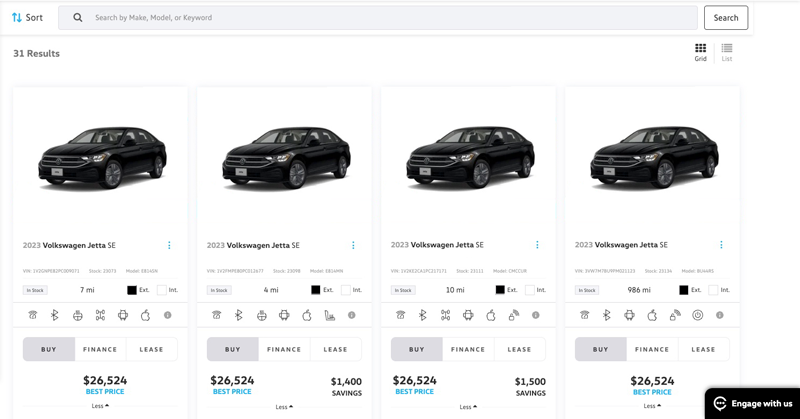The image displays an interface for browsing and sorting a variety of cars. At the top of the image, there is a text that reads "Sort" accompanied by two blue arrows, one pointing upwards and the other downwards, indicating sorting options. Adjacent to this, there's a magnifying glass icon next to a grey search box with the placeholder text “Search by make, model, or keyword,” and a white search button with the text “Search” in black.

The interface indicates that there are 31 results, currently sorted in a grid view format. Displayed prominently on this page are four identical black Volkswagen Jetta SE cars. Each car is listed with a price of $26,524. Some of these listings include potential savings ranging between $1,400 and $1,500. Prospective buyers have the options to purchase, finance, or lease these vehicles.

The listings provide additional details about each vehicle, highlighting exterior and interior colors along with various features. Notable features include Bluetooth connectivity and compatibility with Android Auto and Apple CarPlay. The overall interface is set against a primarily white background with scattered accents of different colors and detailed information about each car.